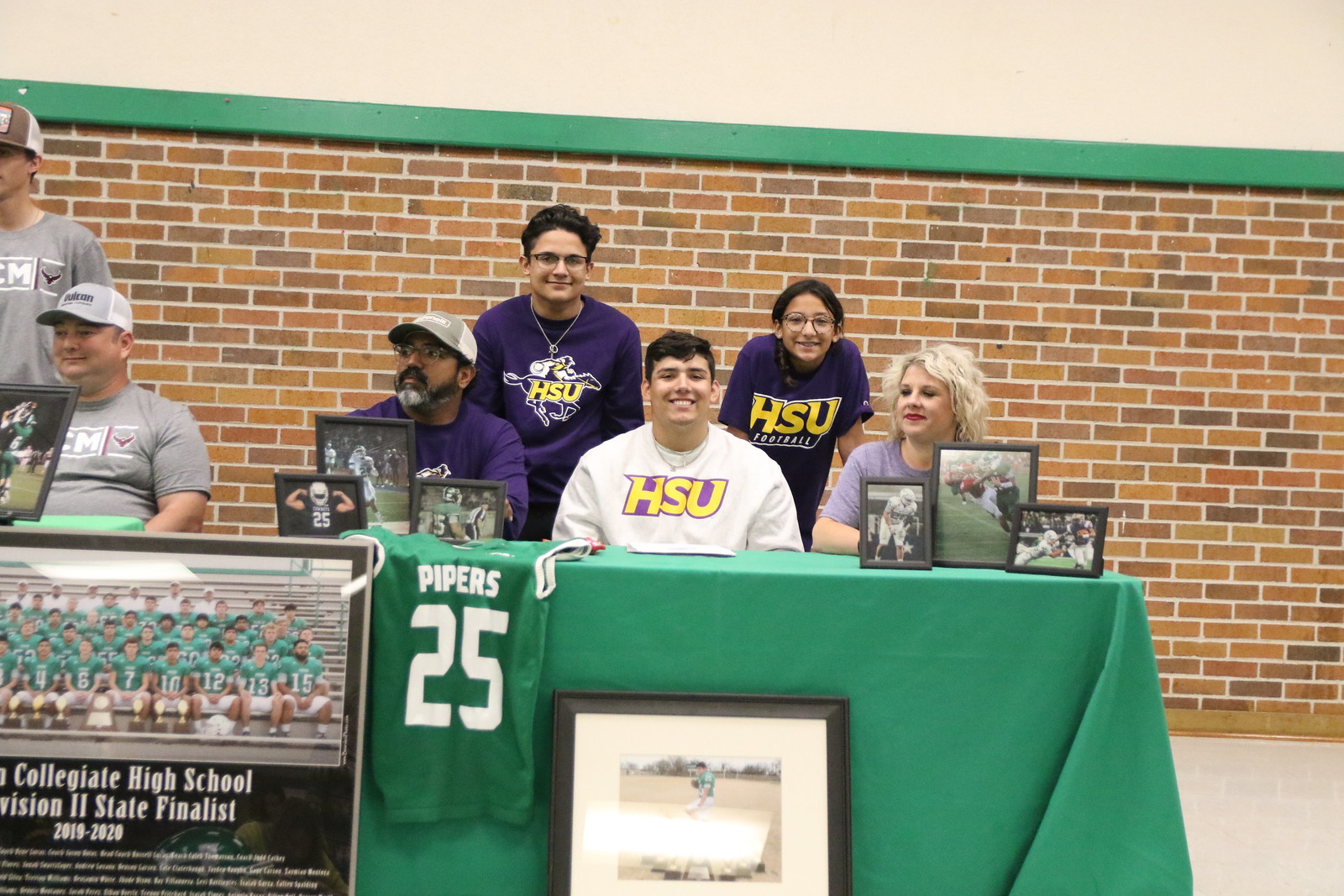In the photo, the setting is an indoor high school recruitment event, with a focus on football. The venue features a tiled floor and a plain brick wall in the background. At the center of the image, a table with a green tablecloth is prominently displayed. Draped over the left side of the table is a football jersey, emblazoned with "Piper, Pipers number 25." In front of the table stands a framed picture of a football player, accompanied by various other photos of football players scattered across the table. Behind the table sit three high school students dressed in HSU school attire. Flanking them are a gentleman on the left and a woman on the right. The image's colors include tan, green, brown, white, gray, purple, black, orange, and red, contributing to a vibrant yet focused scene showcasing a football recruitment activity.